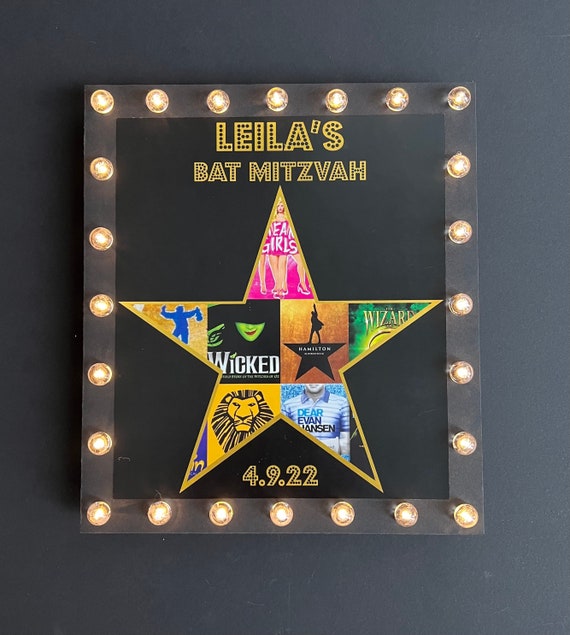The image depicts a framed, light-up decoration on a gray wall, showcasing "Layla's Bat Mitzvah" in bright yellow letters at the top. The frame is black and adorned with glowing light bulbs surrounding a central star outlined in yellow. Inside the star is a collage of popular Broadway show titles such as "Mean Girls" in pink, "Wicked," "Dear Evan Hansen," "Wizard of Oz," "The Lion King" with a black and yellow lion logo, and "Hamilton." At the bottom of the frame, the date "4.9.22" is displayed in yellow numbers. This setup likely serves as a decorative piece for an event, exuding a Hollywood-inspired theme with its illuminated and theatrical presentation.